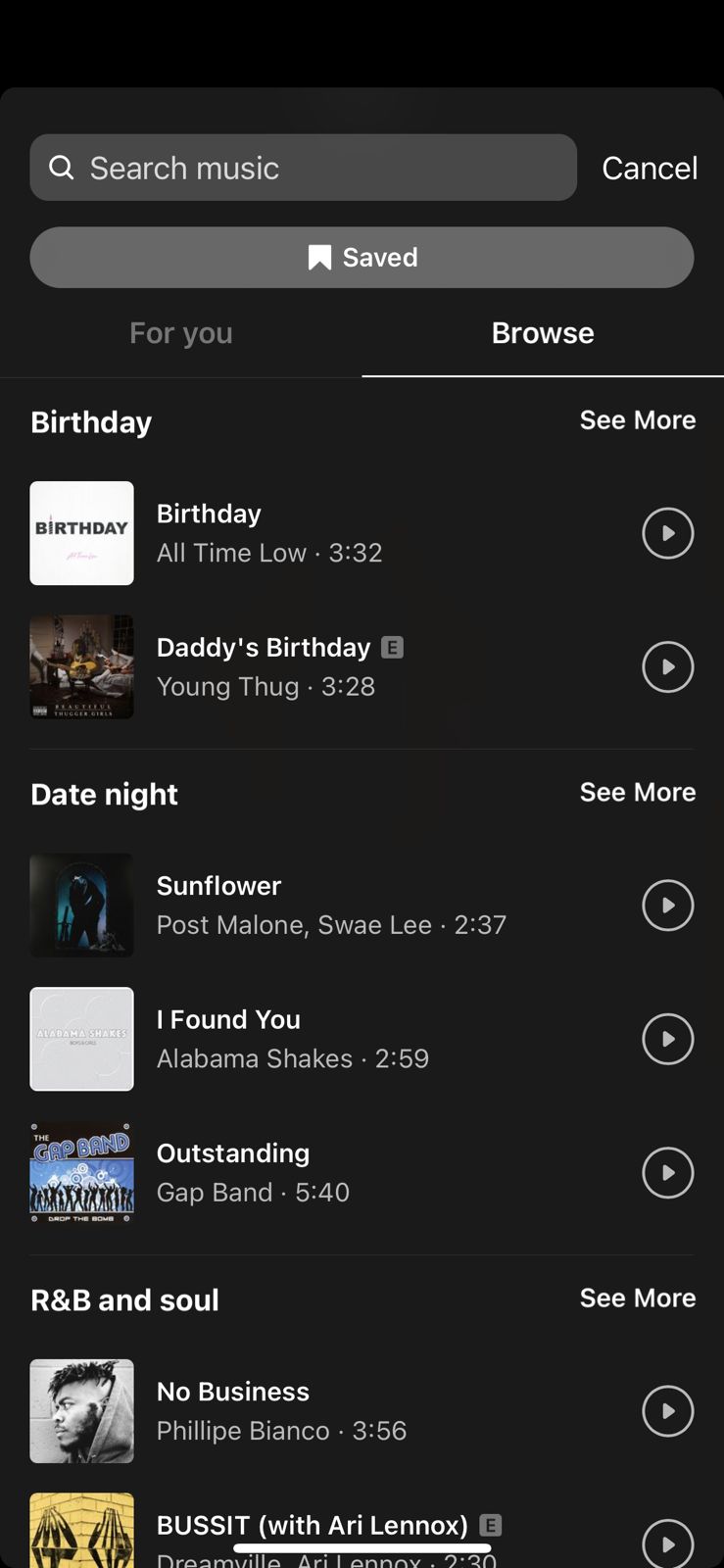The image depicts an interface of a music listening app with a sleek, black background and clean, white text. At the top, there's a search bar labeled "Search Music," accompanied by a "Cancel" button. Just beneath this, there's a "Saved" option.

Two tabs, "For You" and "Browse," are present, with the "Browse" tab currently selected. Directly below this is a title labeled "Birthday," under which two songs are listed: "Birthday" by All Time Low and "Daddy's Birthday" by Young Thug. 

Further down, the header "Date Night" appears, categorizing songs suitable for a romantic evening. Songs in this category include "Sunflower" by Post Malone, "I Found You" by Alabama Shakes, and "Outstanding" by the Gap Band. Below this, the "R&B and Soul" category features tracks like "It's No Business" by Filipe Blanco and "Buss It" by Aerie Lennox.

Each song features its album cover to the left, with a play button positioned at the far right. For instance, the cover for the song "Birthday" features simplistic design: the word "Birthday" in black lettering on a white background.